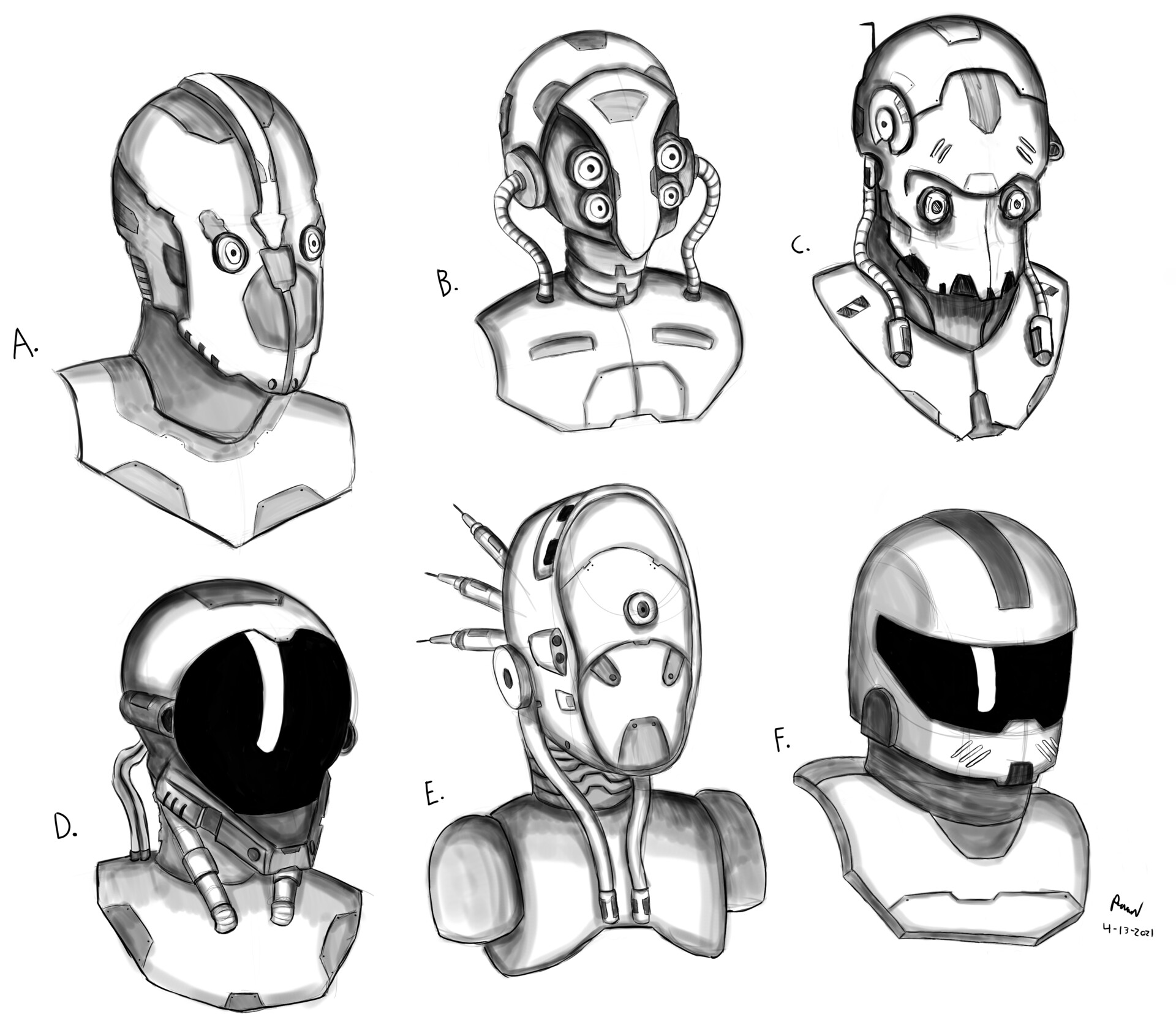This image, displayed on a white background, is a black and white illustration of six different sci-fi helmets, labeled A through F. The layout is structured in a grid format: A, B, and C are in the top row from left to right, and D, E, and F occupy the bottom row. The helmets vary significantly in design and resemble robotic heads, with intricate details highlighting their unique features.

- Helmet A resembles the design of CP-3-0 from Star Wars but rendered in monochrome.
- Helmet B features a lizard-like creature with four eyes and has wires or connectors extending from the sides.
- Helmet C also resembles an animal but is uniquely adapted as a helmet.
- Helmet D has a dark covering over the face, making the person's features indiscernible.
- Helmet E, positioned at the center bottom, has a frowning expression and two eyes.
- Helmet F, similar to helmet D, has a very dark covering over the face, obscuring its features.

All the helmets are intricate and varied, showcasing different types of head coverings and robotic shapes typical of comic book or sci-fi concepts. The small text in the lower corner reads "PAUR 4-13-2021," marking the illustration's date and possibly the artist's initials.